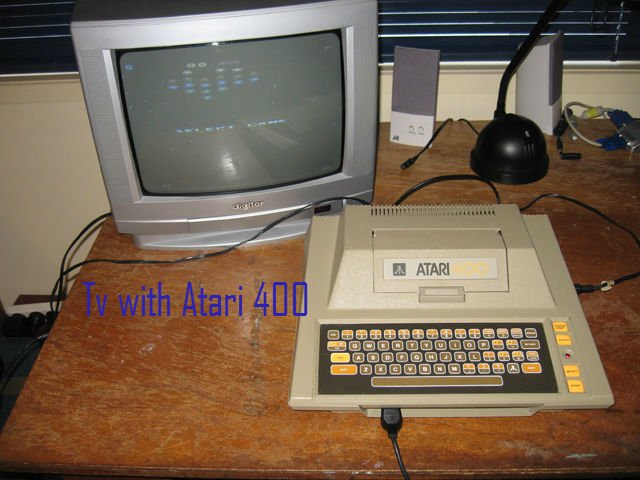In the center of the image is an old-fashioned TV displaying a selection of Atari 400 video games. The television sits atop a brown table. In the top right corner of the scene, there is a set of speakers, larger than any other elements in the image, giving an impression of bulk and prominence in comparison. Near the speakers, there is a fixture with black cables and strings hanging down.

On the bottom right, an Atari 400 console, characterized by its off-white plastic casing, is visible. The console features a keyboard layout with numerous keys, most notably a QWERTY setup and functional rows marked by labels such as "ASDF." Noteworthy are the yellow function keys positioned to the right. There is also a cable connected to the Atari console.

The screen on the TV is vibrant, showcasing a colorful game selection interface. To the left of the table, multiple cables can be seen plugged into a power outlet, contributing to the vintage and electronic feel of the setup.